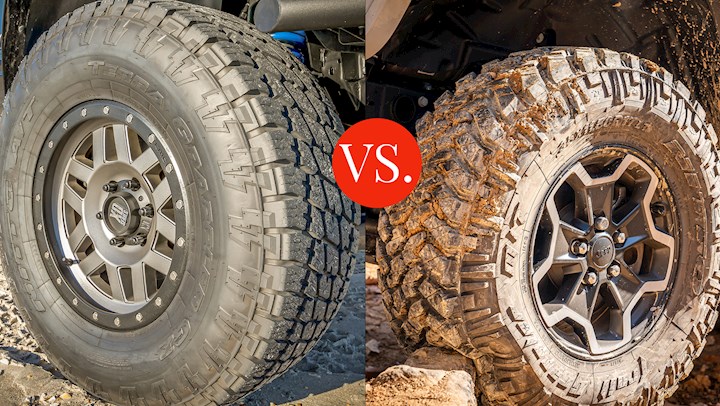In this promotional image for heavy-duty, all-terrain truck tires, two comparative photos are displayed side-by-side against a potentially beachy terrain with a mix of sand, dirt, and cement. The left image showcases a clean, brand-new tire fixed by six bolts, featuring pristine deep, rugged treads and shiny hubcaps. This tire retains much of its original black color, exuding durability and freshness. In stark contrast, the right image depicts a tire in action within a muddy, rocky environment. The tire is encrusted with dirt, mud, and small rocks, further emphasized by the dirt flying off in the image's top right corner. This tire is mounted with five bolts and is notably compressed against a significant rock or cement piece, illustrating its flexibility and the rough conditions it can endure. In the background, the blue shocks of the trucks and part of the chassis are visible, highlighting the rugged capabilities of these tires amidst challenging terrains. Text reading "VS." separates the two images, underscoring the comparison between the pristine and the rugged states of the tires.